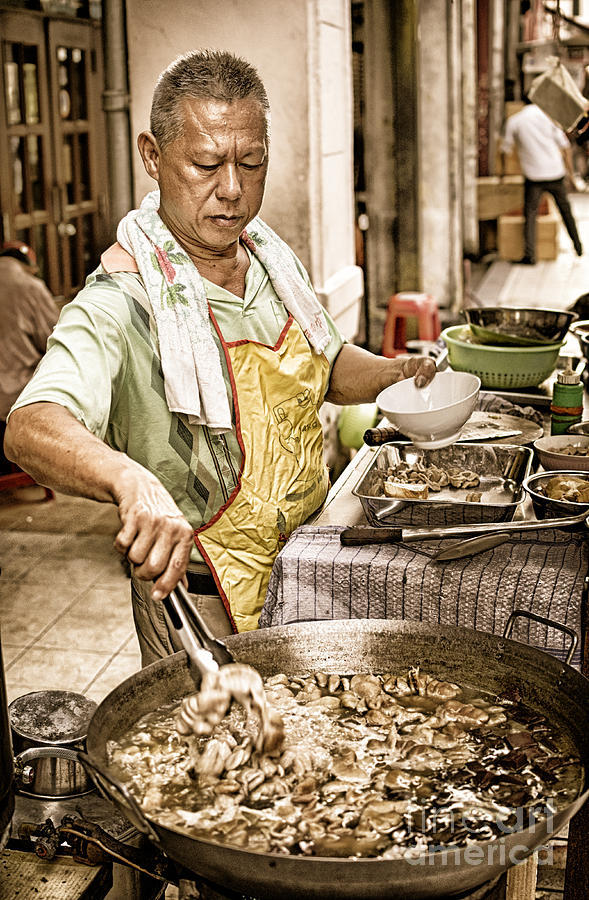In a captivating sepia-toned image that evokes the essence of street food culture, an East Asian man stands at the forefront, deeply engrossed in his culinary craft. He wears a light green collared shirt and a striking yellow apron with a red outline. Draped over his neck is a light green and white patterned dish towel adorned with red and green leaves and flowers. With short, spiky, grayish hair and dark skin, he skillfully maneuvers a pair of metal tongs in his right hand to stir food in a gigantic metal wok, while his left hand holds a white, empty bowl, poised to serve his creation. The bustling scene extends beyond him, revealing a semi-busy alleyway with street and buildings and additional food and utensils laid out in front of him, including a strainer and an orange stool. A second man, wearing black pants and a white shirt, is partially visible in the background. A "Fine Arts America" watermark discreetly marks the bottom right corner, affirming the image's artistry and authenticity.